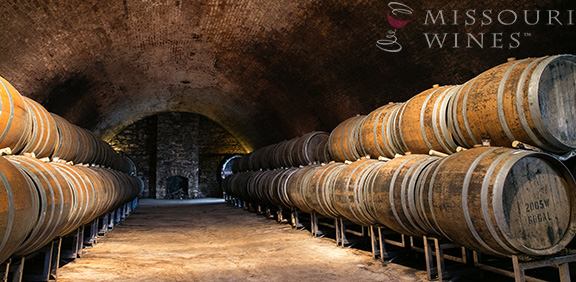The photograph depicts a large underground wine cellar with an arched brick ceiling, showcasing numerous wooden wine barrels stacked in double layers on both sides of a long corridor. The barrels, set on metal stands, appear weathered and some bear stenciled markings like "2005 W 60 gal," indicating their volume and possibly their fill date. The aisle stretches toward an old, disused stone fireplace at the far end, which is flanked by some ambient wall lighting. Prominently visible in the top right corner of the image is a transparent light gray text overlay reading "Missouri Wines," accompanied by a logo featuring a stylized spiral line and a hint of red, suggesting a glass of red wine. The floor beneath the barrels is a lighter beige color, contrasting with the dark browns, blacks, reds, whites, and grays that form the rich palette of the scene. The entire setting exudes an atmosphere of historical charm and diligent craftsmanship characteristic of a Missouri wine cellar.